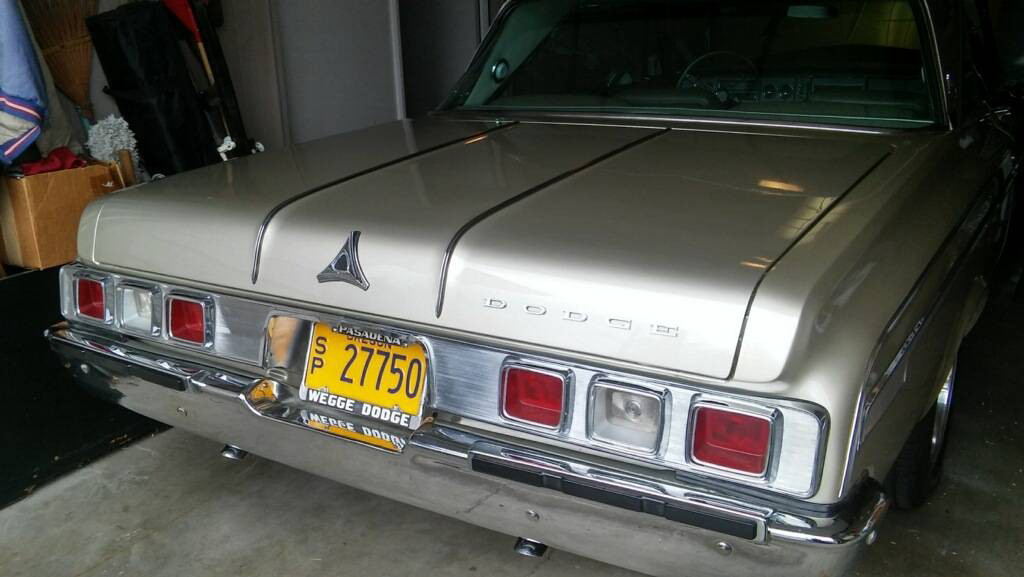This is a detailed photograph showcasing the rear end of a vintage, light grey Dodge car parked in a cluttered garage. The vehicle features a distinctive yellow Oregon license plate with the registration SP27750, framed by a holder inscribed with "Wedge Dodge." The license plate is centrally positioned on the trunk, flanked by two sets of three square taillights. Each set comprises a red light, a clear light, and another red light. The bumper is shiny silver metal, and silver embellishments accentuate the sides and taillights of the car. Although the image is somewhat dark, you can glimpse the back window and notice the garage's clutter, including storage items like boxes and a suitcase on the left side of the car. The overall impression is one of a wide, boxy rear end characteristic of a classic Dodge.